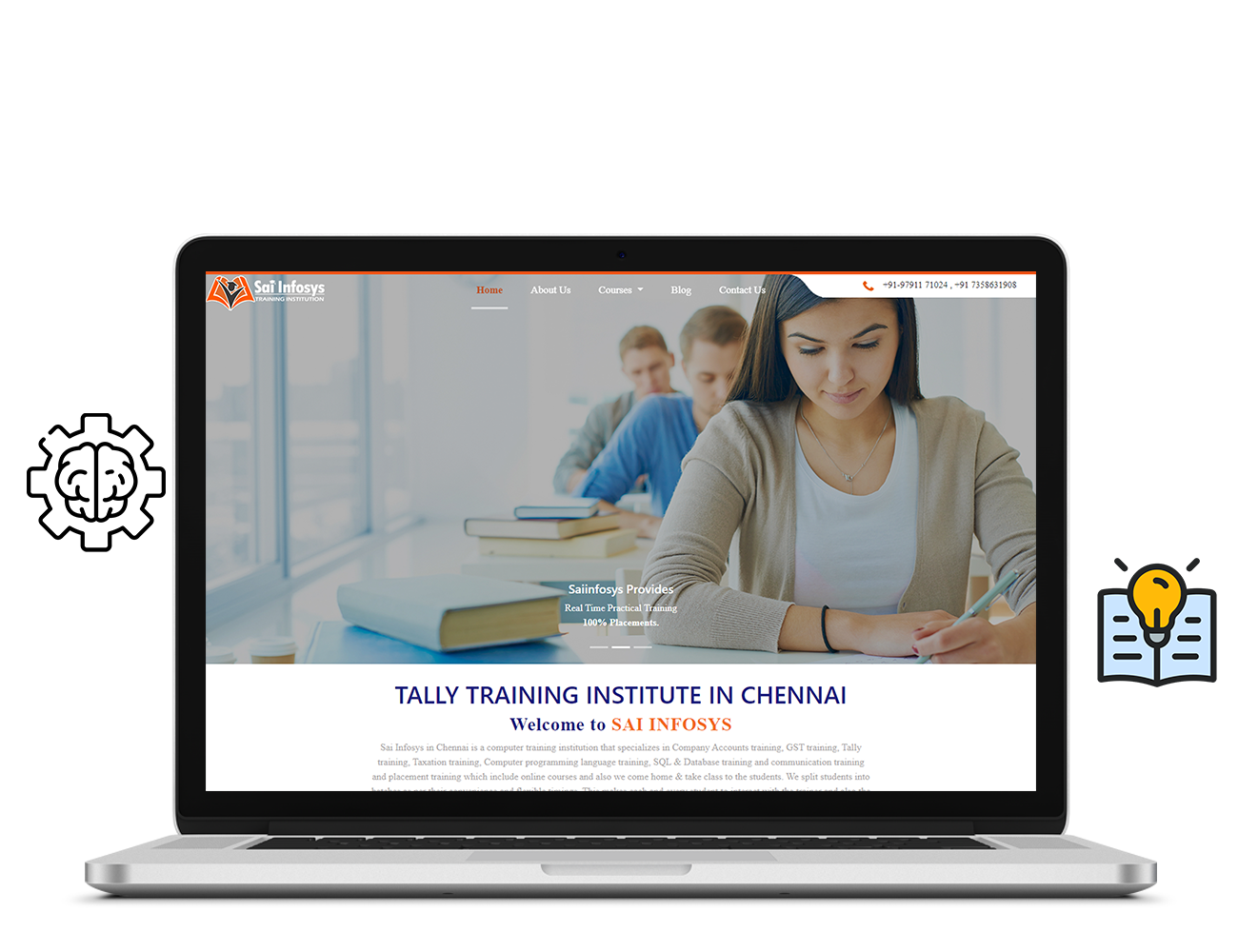A modern laptop rests on a pristine white surface, set against a clean white background, creating a minimalistic and sleek setting. The laptop screen displays a webpage from SALSAINFOSYS Training Institution. 

The page background shows three individuals, a woman followed by two men, each diligently working at desks arranged one behind the other. 

In the upper left corner of the screen, a logo reads "SALSAINFOSYS Training Institution." 

A navigation bar spans the top of the page, featuring links titled Home, About Us, Courses (with a drop-down menu), Blog, Contact Us, and Phone. Two phone numbers are listed prominently: +91 97911 71024 and +91 73586 31908.

A prominent middle-section banner declares, "SALSAINFOSYS provides real-time practical training with 100% placements."

Beneath this, white text on the same background states, "Training Institute in Chennai."

The bottom of the screen welcomes viewers with the text, "Welcome to SALSAINFOSYS," followed by a brief description, "SALSAINFOSYS in Chennai is a computer training institute."